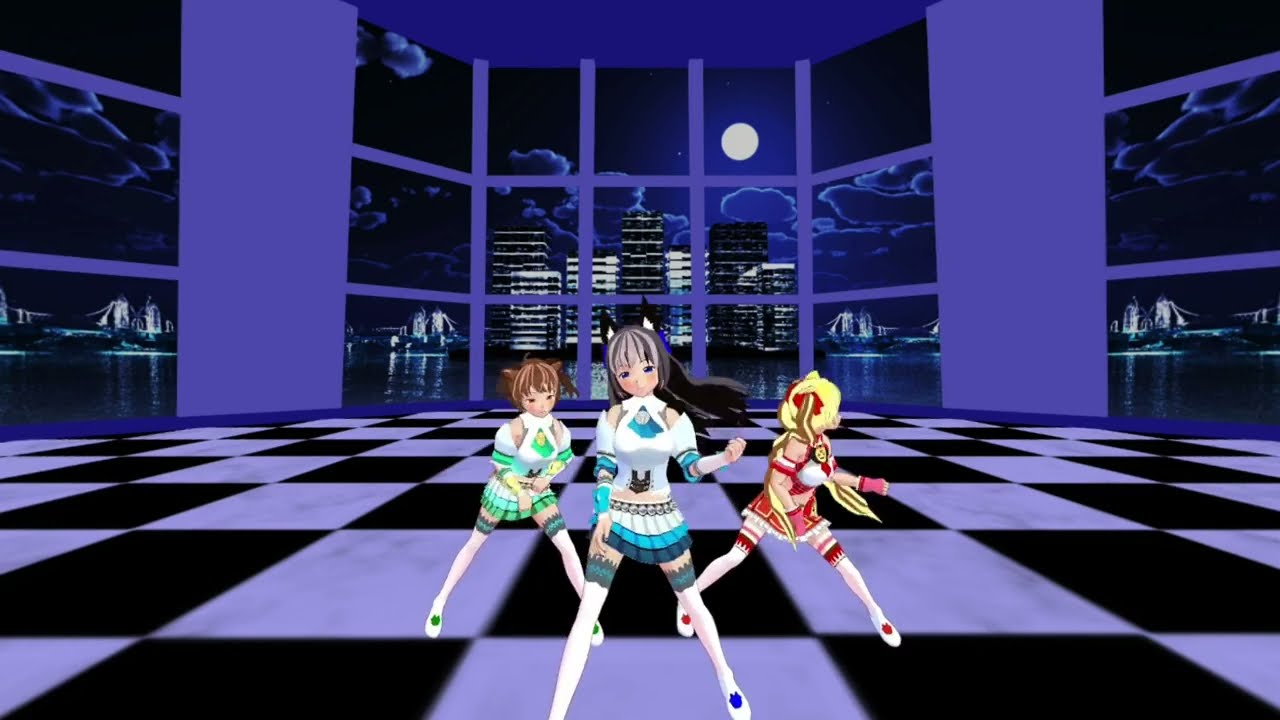Here is a detailed and cleaned-up caption for the image:

"The scene portrays an animated Japanese-style image of three female dancers on a black and white checkerboard floor. The central dancer, slim with an animated Japanese face, wears a mini skirt, white socks, and an outfit with white and bluish trim. To her left is another dancer, characterized by her yellowish hair and a red and white outfit, with a less human, possibly pig-like head turned to the left. On the right is a third dancer in a light green and white shirt, positioned slightly behind the central dancer. They all appear to be dancing in this spacious room. Large floor-to-ceiling windows with light purple frames line the back wall, revealing a nighttime scene outside. A large moon hangs in the sky, illuminating a river that runs past the room, with a silhouette of towering skyscrapers composing the cityscape on the opposite shore."